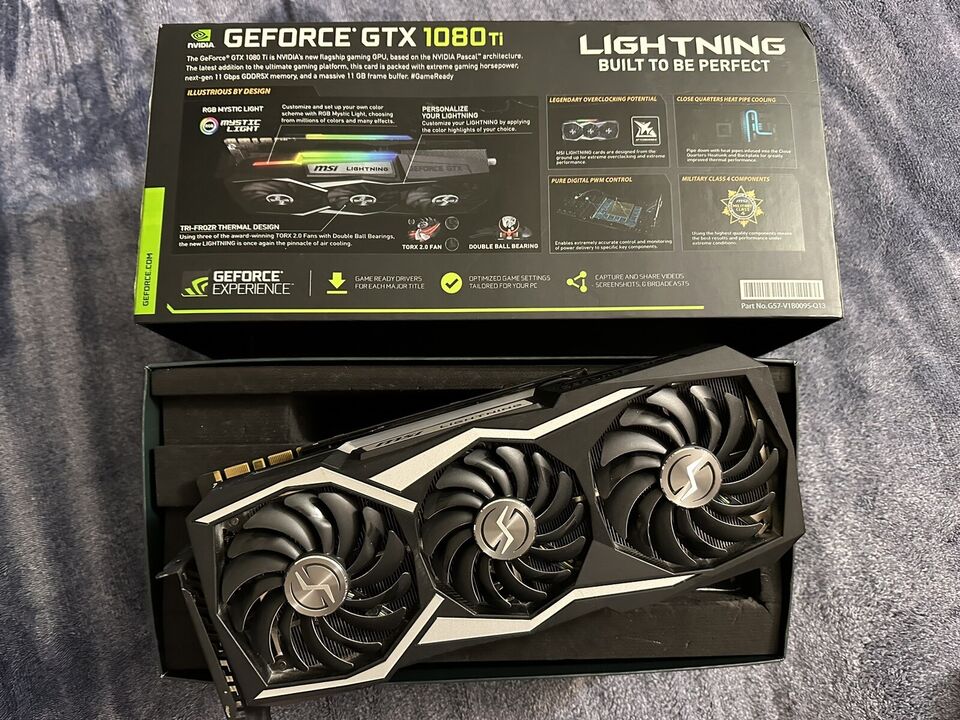The image shows a GeForce GTX 1080 Ti graphics card made by MSI, prominently displayed with both its box and the card itself in view. The black box is positioned at the top and includes comprehensive information and a colorful design, prominently featuring the phrases "lightning built to be perfect" and "GeForce Experience," along with the NVIDIA and MSI logos. The box also includes a QR code at the bottom right. Below the box, the graphics card rests diagonally on black foam packaging, which snugly fits inside the box. The card's black and silver design is highlighted by three centrally silver-lined fans, each fan containing densely packed, curvy, thin black blades. The environment in which the photo is taken includes a towel in the background, confirming an indoor setting. The box art reflects the card's design, showing off RGB features and emphasizing its premium, high-performance build.